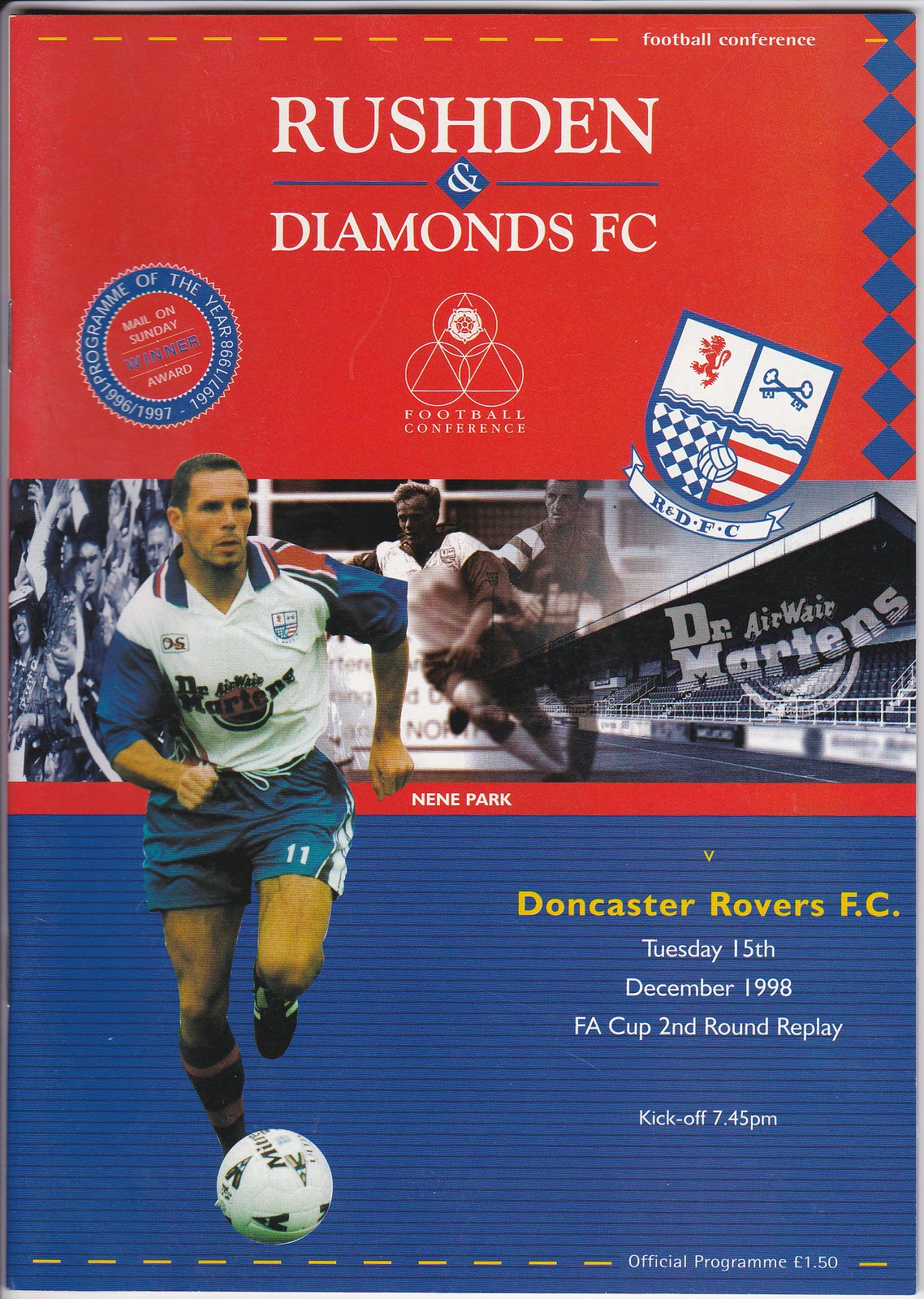This image is an advertisement for a soccer game featuring Rushden and Diamonds FC and Doncaster Rovers FC. The top third of the image has a red box with white, all-caps font that reads "Rushden and Diamonds FC." Below this, there's a circle highlighting "Program of the Year 1996-1997 and 1997-1998." Vertically down the right-hand side, you can see blue diamond shapes. At the center of the page, there's a red bar with white font that states "Nene Park." Below, in a blue section, it reads "Doncaster Rovers FC" in yellow font, with details of the match in white font: "Tuesday, 15th December 1998, FA Cup Second Round Replay, kickoff 7:45 p.m." The background of the middle of the image displays people playing soccer, spectators, and a stadium. Overlaying this background on the left-hand side from the middle to the bottom, there is an image of a soccer player in a white jersey with red and blue accents, blue shorts, and black shoes, running and about to kick a soccer ball.